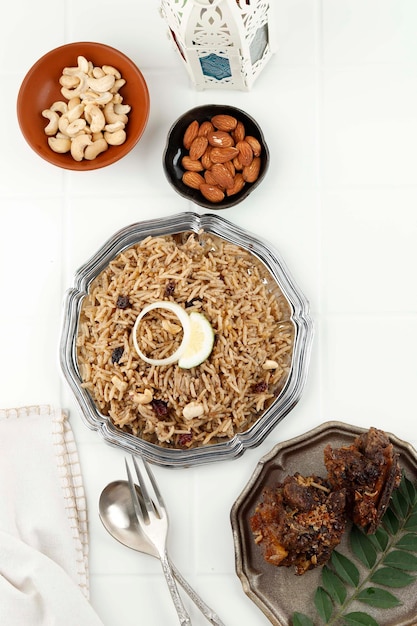This overhead photograph depicts a beautifully arranged meal on a bright white tiled surface. In the center of the image, a large ornate silver platter holds a dish of long-grain basmati rice, tinged brown from a savory sauce. The rice is studded with various ingredients, which might include nuts or dried fruits, and features a central garnish of a lemon wedge and a ring of white onion. At the top of the photo, a white decorative candle holder with intricate cutouts adds an elegant touch. Below it, on the left, there is an orange bowl filled with cashews, and to the right, a black bowl containing whole almonds with their skins on.

To the bottom right of the main dish, a smaller grayish metal plate displays two dark, possibly fried, chunks of meat or date balls, accompanied by a green sprig, which could be either mint or a fern-like leaf, serving as a garnish. Positioned carefully to the left of this smaller plate are a metal fork and spoon, resting beside a neatly folded white cloth napkin with decorative stitching along the edges.

The entire setting creates a harmonious blend of rich textures and earthy tones, set against the pristine white backdrop, emphasizing the thoughtful presentation of the meal.